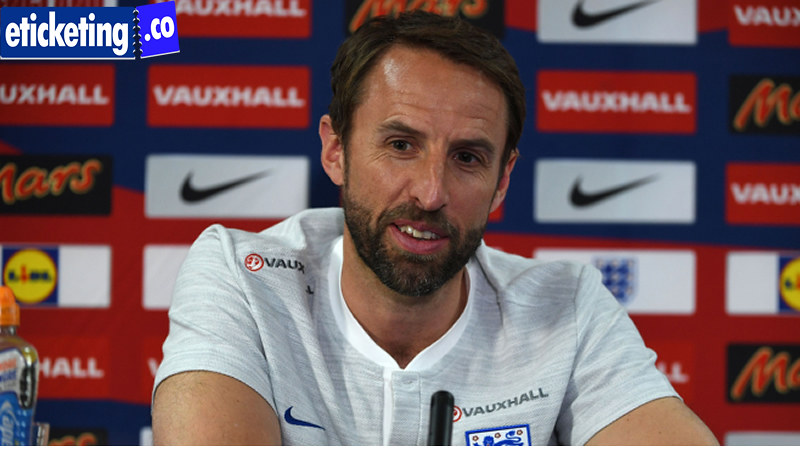A man with black hair and a black beard, wearing a light grey t-shirt adorned with two Voxhall logos, is seated on a stage, presumably following a sporting event. The backdrop is covered with recurring logos, including those of Voxhall, featuring a red triangle, Nike with a white rectangle, and Mars within a black rectangle, among others that are less discernible. He is positioned centrally in the image with a microphone in front of him, appearing to look down towards the press or audience, likely answering questions in what seems to be an indoor setting for a pre-game or post-game press conference. An eTicketing.co watermark is visible in the upper left corner, depicted in white font set against a blue background with varying shades. The scene is underscored by the presence of multiple advertisements, reinforcing a professional and media-centric environment.